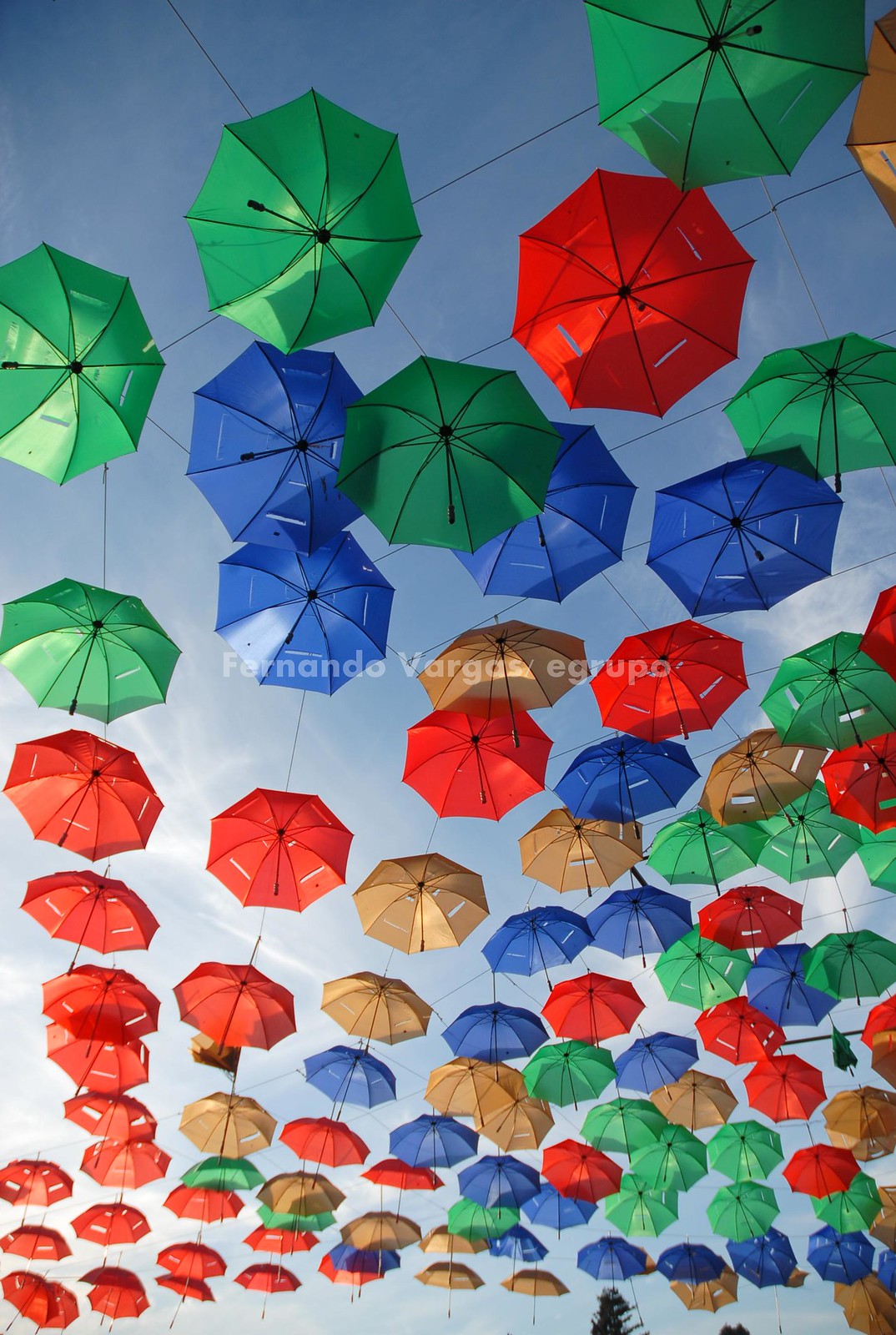Against a gradient blue sky that transitions from medium blue at the top to a light blue at the bottom, an array of colorful umbrellas appears to be suspended mid-air, creating a visually striking scene. The umbrellas, which come in shades of red, green, medium blue, and a brownish-yellow, are meticulously strung up by thin, barely visible wires, giving the impression that they are floating. The umbrellas are uniformly designed and fully open, with many seemingly turned upside down. This artistic display, with about 40 to 80 umbrellas in total, bathes in sunlight that streams through their canopies. Below this mesmerizing installation, a couple of evergreen trees peek into the frame, adding a touch of nature to the surreal composition.